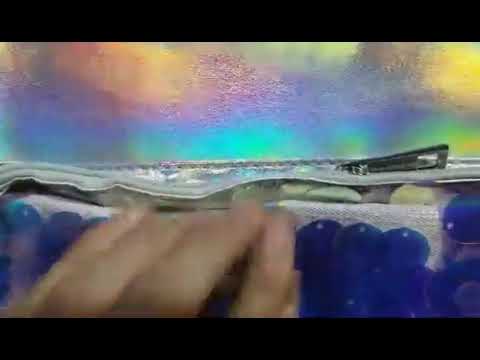In this blurry, letterboxed image, a person's left hand, identifiable by four visible fingers and part of a thumb, is reaching upwards to grasp an indeterminate, shiny, and iridescent object. The hand appears to rest upon or interact with a cluster of rounded blue objects, resembling gemstones or aquarium rocks, numbering around 20 to 30. To the immediate left and right of the hand, the blue objects continue in a strip, creating an intriguing contrast against the more vivid elements in the background. The upper part of the image features a background awash with a blend of iridescent, faded hues—purple, blue, yellow, lime green, and pink—melding together in a dreamlike swirl that might evoke an impressionistic painting of a choppy ocean or a vividly colored sky. Behind the hand, a white object, possibly resembling a purse with a zipper, further muddles the scene. The overall composition is quite hazy, making it challenging to decipher the specific elements clearly.